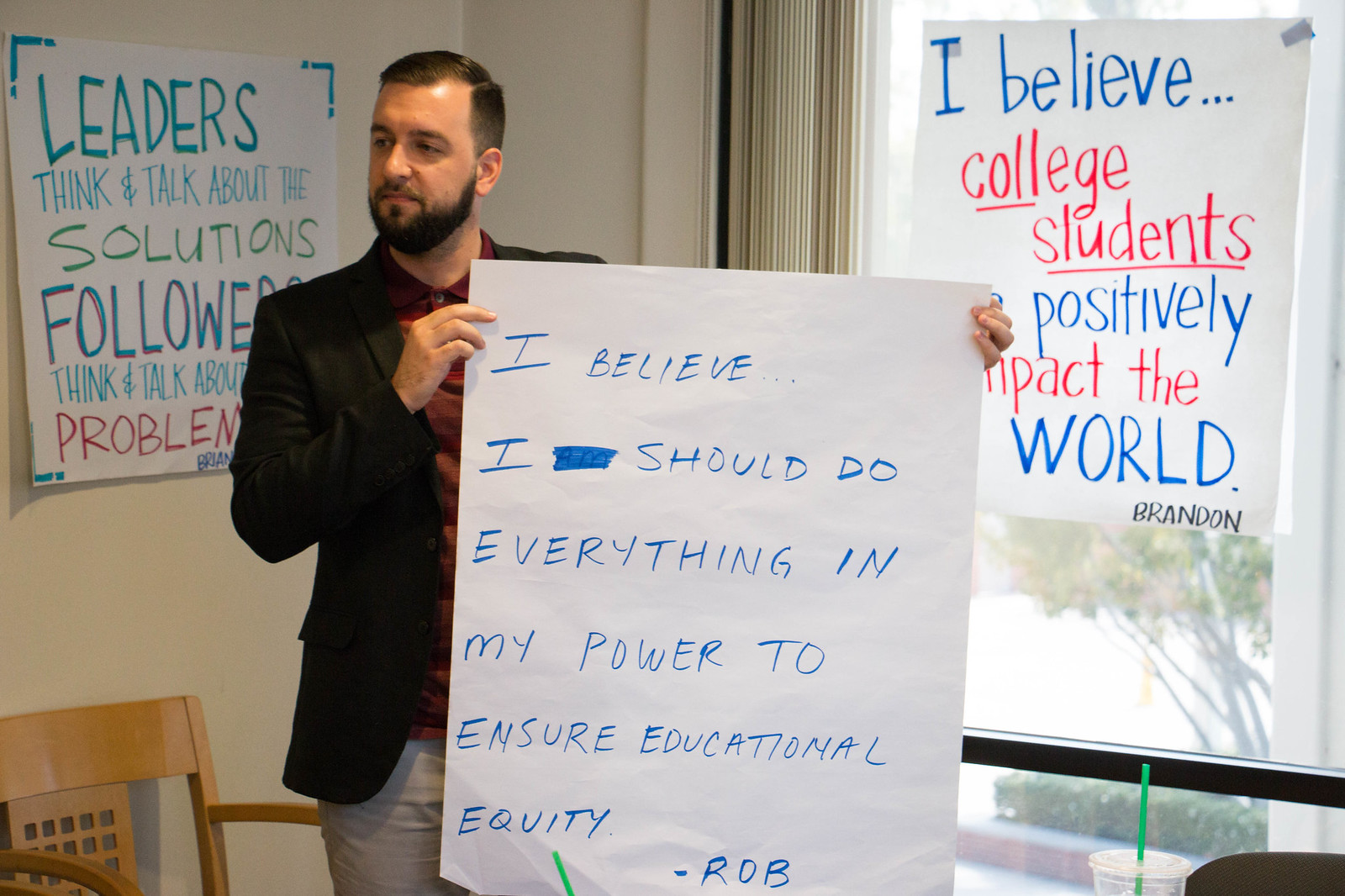In the image, a man wearing a black suit jacket over a maroon polo shirt and beige pants is holding a large white paper with handwritten text in blue ink that reads, "I believe I should do everything in my power to ensure educational equity. - Rob." The man has short, neatly-combed brown hair with the sides buzzed and a black beard along his jawline. He is standing inside a room with a white wall behind him. To his right, there's a window with white blinds, and a white piece of paper stuck on it saying, "I believe college students positively impact the world. - Brandon." On the left wall, there's another large white piece of paper that reads, "Leaders think and talk about the solutions. Followers think and talk about problems." A wooden chair is visible on the lower left, and on the lower right, there's a clear cup with a green straw, likely a Starbucks cup, along with a black chair. The photo captures a setting that appears to be educational, hinting that the man could be a teacher or a student involved in a classroom activity focused on inspirational messages.